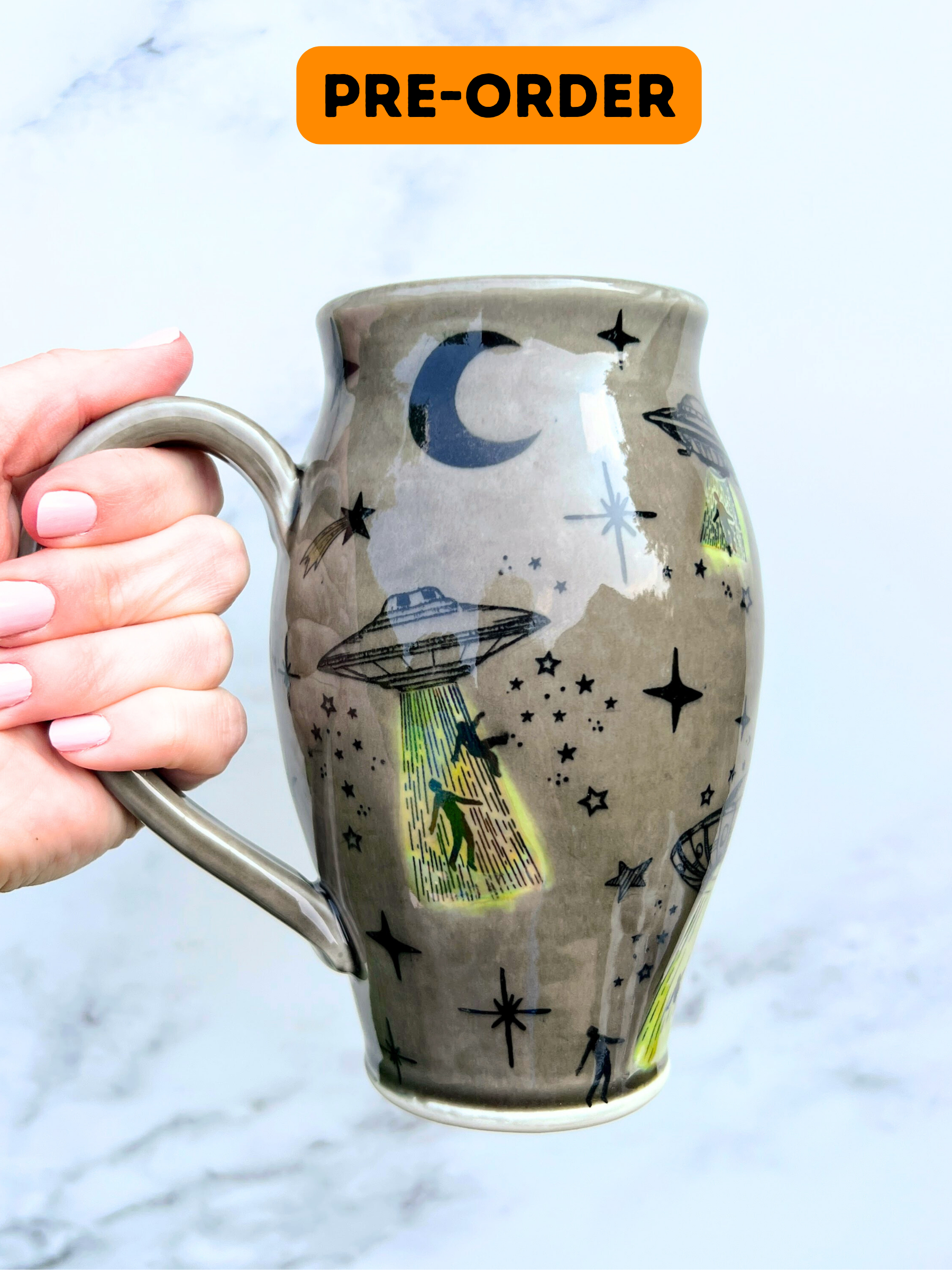In the photograph, a light-complexioned hand with pink painted nails is holding a uniquely shaped mug, which appears as half of a stylized heart. The background is a softly blurred light gray marble texture. The mug itself is a glossy greenish-gray color adorned with various black silhouetted designs. These designs include a crescent moon at the top, scattered stars in both cross and five-pointed shapes, and three visible flying saucers positioned on the left, top right, and bottom right. Each flying saucer projects beams of black, yellow, and green light beneath them, showing silhouetted figures being pulled into the spacecraft. The overall design exudes a strong sci-fi movie and space theme. At the top of the mug, there's an orange rounded rectangle with thick black text that reads "pre-order."